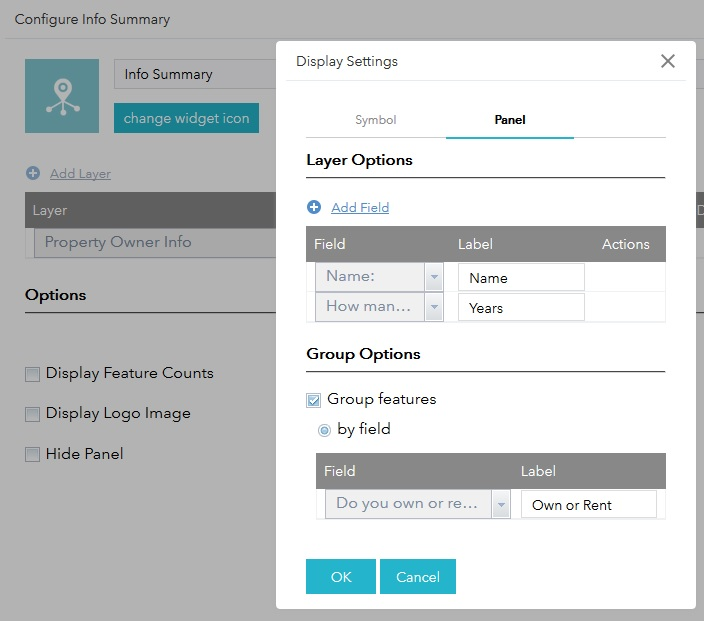The image is a detailed screenshot from an unidentified website, featuring a user interface divided into two main sections: a grayed-out background area and a prominent white pop-up window.

The grayed-out background area contains multiple menu options that can be read despite being de-emphasized. These options are listed as follows: "Configure Info Summary," "Info Summary," "Change Widget Icon," "Add Layer," "Layer," "Property Owner Info," "Options," "Display Feature Count," "Display Logo Image," and "Hide Panel."

On the right side, the white pop-up window titled "Display Settings" occupies a significant portion of the screen. Within this window are several sub-sections and interactive elements:

- **Symbol and Panel**: The term "Panel" is highlighted, indicating it has been selected.
  
- **Layer Options**: Includes an option to "Add Field."

- **Field Settings**: 

  - **Field Name Options**: Lists fields such as "Name," "How Many," "Label," "Name," and "Years."
  - **Actions and Group Actions**: Includes a checkbox, which is selected, for grouping features.
  - **Field Ownership**: Shows a selected checkbox for "Buy Field" and includes a field labeled "Do You Own or Rent," with a corresponding label of "Own or Rent."
  
- **Controls**: At the bottom left, the pop-up window provides two turquoise buttons — "OK" and "Cancel," written in white letters.

This image is entirely textual, devoid of any photographs, people, animals, plants, flowers, trees, or vehicles.